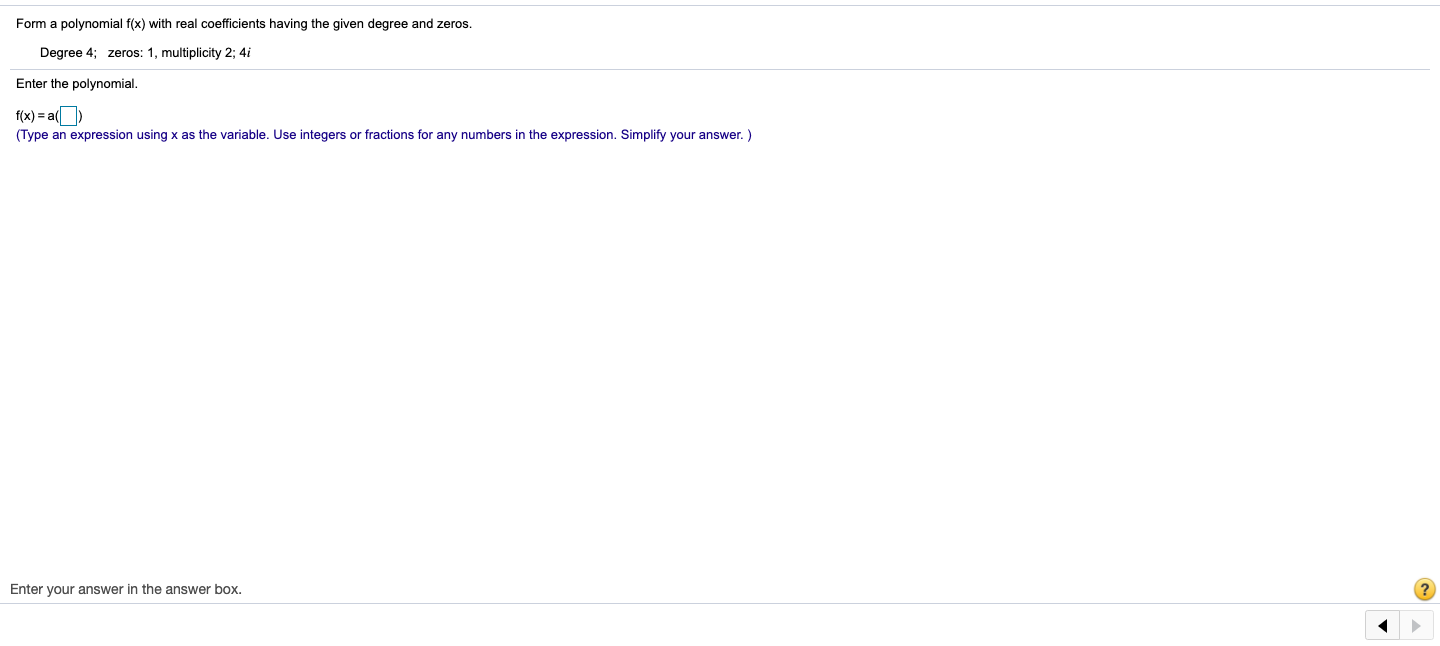This is a detailed screenshot of a mathematics website interface designed for solving polynomial problems. The page features a clean, all-white background with a specific instructional prompt in black text: "Form a polynomial, \( F(x) \), with real coefficients having the given degree and zeros." Following this instruction, it specifies that the degree of the polynomial is 4, the given zeros are \( 1 \) with a multiplicity of 2, and \( 4i \).

Below this, there's a directive to enter the polynomial in the format \( F(x) = A \), with a blank input box provided for the user to fill in the polynomial expression. An important note appears in blue text, guiding users to "type an expression using \( x \) as the variable, use integers or fractions for any numbers in the expression. Simplify your answer."

Underneath this instruction, the text "enter your answer in the answer box" is displayed in black, along with a yellow question mark icon to the right, suggesting that additional help or explanation is available.

At the bottom of the screen, navigation arrows are present. A black arrow pointing left indicates the option to go back, while a grayed-out arrow pointing right suggests that the forward option is currently unavailable.